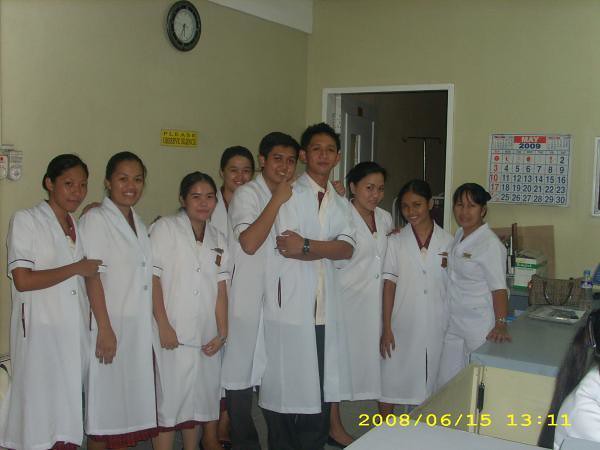This image captures nine dark-skinned individuals, likely medical staff, posing in what appears to be the lobby of a healthcare office. The room has yellow walls and a visible doorway framed in white in the background. A calendar on the wall, with a red background and white markings, indicates May 2008. Positioned near the calendar is a tall individual in the front, with a male standing right behind him, his arm resting on the tall man’s shoulder. Surrounding them are seven other individuals arranged in tiers: four behind the man with the hand on the shoulder and three behind the tallest man. They are all dressed in white lab coats that reach their knees. All of the women have their hair pulled back, and the men, who have short brown hair, give the impression of being quite young. There's a partial view of an additional individual sitting at a high counter, likely the check-in desk, on the bottom right corner of the image. The photograph has a time and date stamp in the bottom right corner, marked in yellow font, noting "2008/06/15 13:11." The specific details of their faces are difficult to discern due to the image being somewhat small and blurry, making it challenging to determine their exact geographical or ethnic origins.